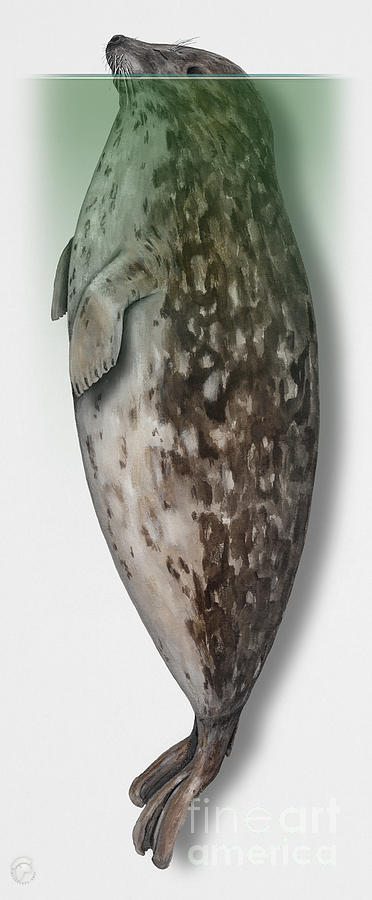The image depicts a detailed, fine art representation of a seal, created by Fine Art America. The seal is upright, with its head and shoulders protruding above the water, which has a greenish tint. The seal has a brown mottled back, with a gray and whitish-gray belly marked with brown splotches. Its head is adorned with numerous whiskers, a black nose, and black eyes that peek above the water's surface. The seal's front flippers are folded across its belly, while its back flippers extend downward. The background above the waterline transitions to a white hue, enhancing the realism of the water surface. Text reading "Fine Art America" appears in white at the bottom right corner of the artwork. Overall, the intricate details and color variations emphasize the lifelike yet artistic quality of the image.